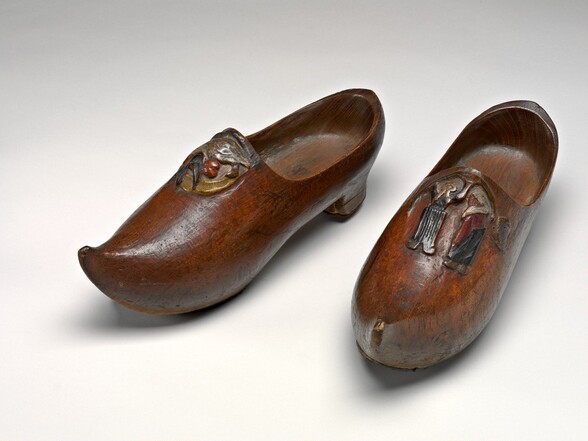This photograph showcases a pair of handcrafted wooden clogs set against a gradient background that transitions from white to darker gray, reminiscent of a museum documentation setting. These dark reddish wooden shoes have a polished surface that reflects light, enhancing their shiny appearance. Each shoe features a pointed, upward-curving toe akin to a canoe's prow, and a carved-out heel measuring approximately an inch high. Ornate carvings and etchings decorate the top, including a distinct design of a man and a woman in heavy clothing on one shoe, and an intricate depiction of an animal or plant on the other. Additional gold ornamentation with a red dot and curves adorns the tongue area, though some of this metal detailing appears slightly rusted. The shoes are positioned at an angle, pointing towards the lower left corner, with shadows cast around them, highlighting their three-dimensional form and compact size.